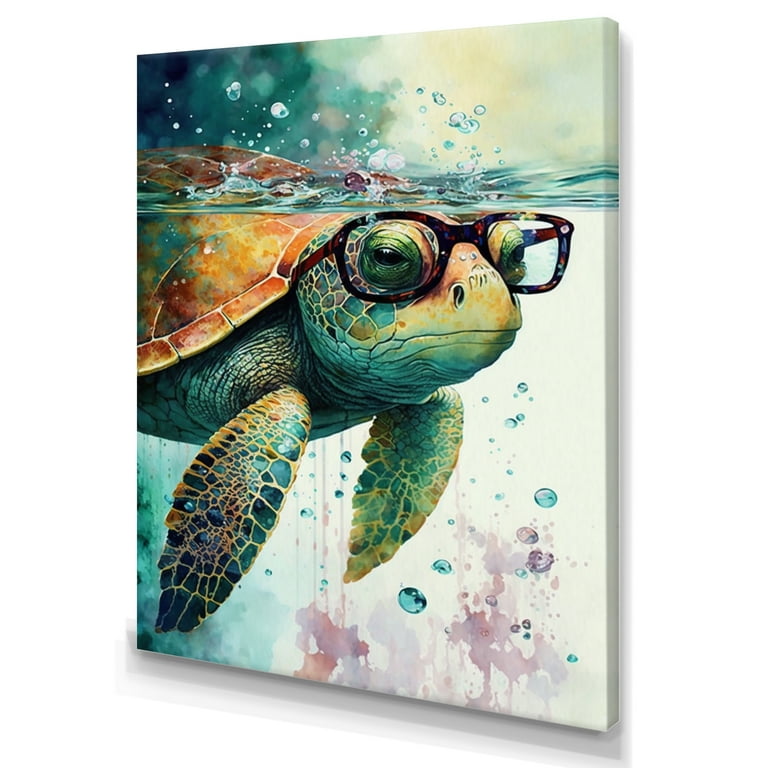The image is a professionally illustrated, frameless canvas print featuring a whimsical sea turtle underwater. The thin, stretched canvas is adorned with a colorful depiction of a sea turtle, whose head and shell partially break the water's surface, creating a playful blend of underwater and above-water elements. The turtle wears large, black tortoiseshell glasses, adding a charming and quirky touch to the piece. His eyes are both black and green, looking off to the right with a wise expression.

The turtle's carapace is a brown mottled with yellow and blue, contributing to the sandy-brown appearance, and his fins are painted in a blend of turquoise and lighter green, with tan outlines that highlight the scaliness of his skin. Sunlit water droplets are illustrated spraying above him, while beneath the surface, the water is suggested by a sparse but vibrant mix of watercolor blues, purples, and pinks that mimic underwater plants and bubbles.

The upper part of the image hints at a blue sky, while the background is primarily white with artistic turquoise bubbles and ghostly watercolor shapes, adding to the dreamy underwater ambiance. This delightful and colorful painting, rich with imaginative details, seems perfectly suited for a child’s room.